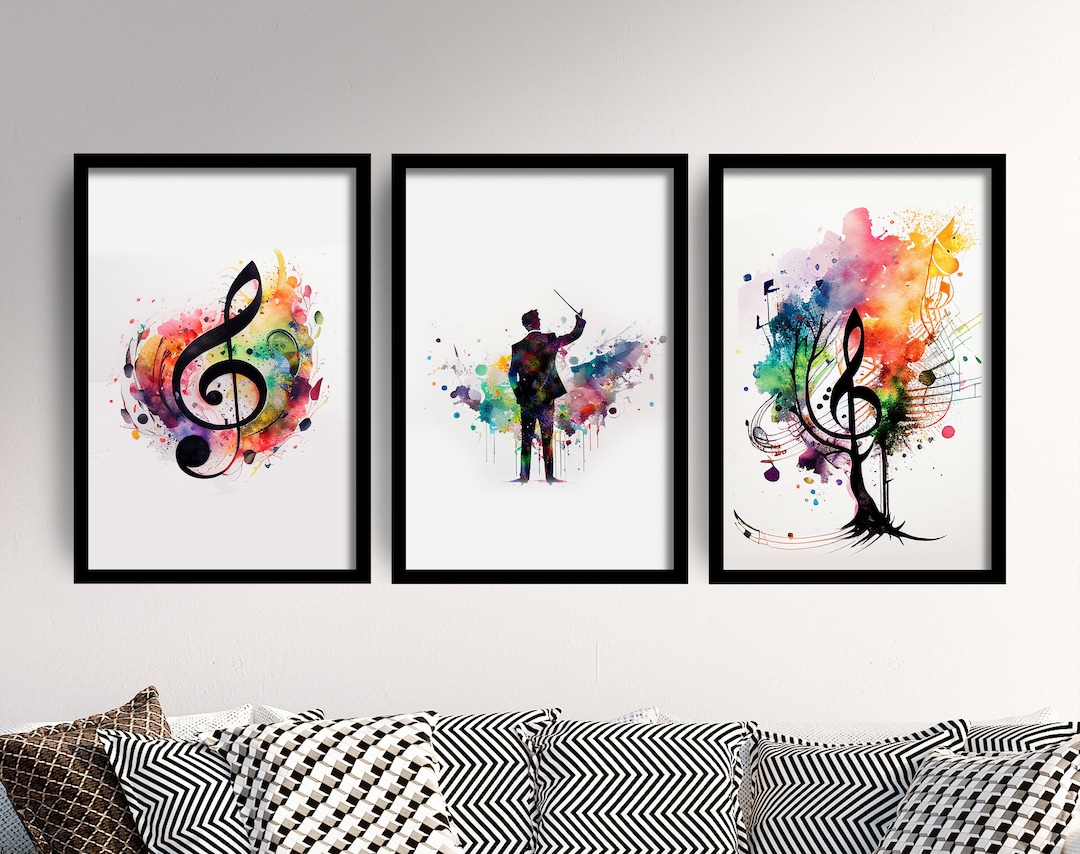The image depicts a modern room with a stark white wall adorned with three black-framed posters. Each poster features a white background with colorful, artistic elements related to music. The left poster showcases a black treble clef against a backdrop of vibrant, multicolored paint splatters including red, yellow, blue, green, orange, and purple. The center poster features a partial silhouette of a conductor, identifiable by a white collar and a conducting baton, enveloped in splatters of yellow, blue, green, purple, and red. The right poster, depicts a black treble clef morphing into a tree with branches, intertwined with paint splashes in green, blue, yellow, red, orange, and pink, along with floating musical notations. 

Below the posters, a couch or daybed is situated, adorned with a variety of eight pillows. The pillows predominantly feature black and white geometric patterns, including zigzag stripes reminiscent of Greek vase designs. The third and eighth pillows display a more intricate pattern of overlapping squares in white, gray, and black. One notable exception is a brown pillow on the left, adorned with a lighter brown diamond design. The modern aesthetic of the room is highlighted by the harmonious blend of monochromatic and multicolored elements, coming together to create a visually stimulating yet cohesive decor.